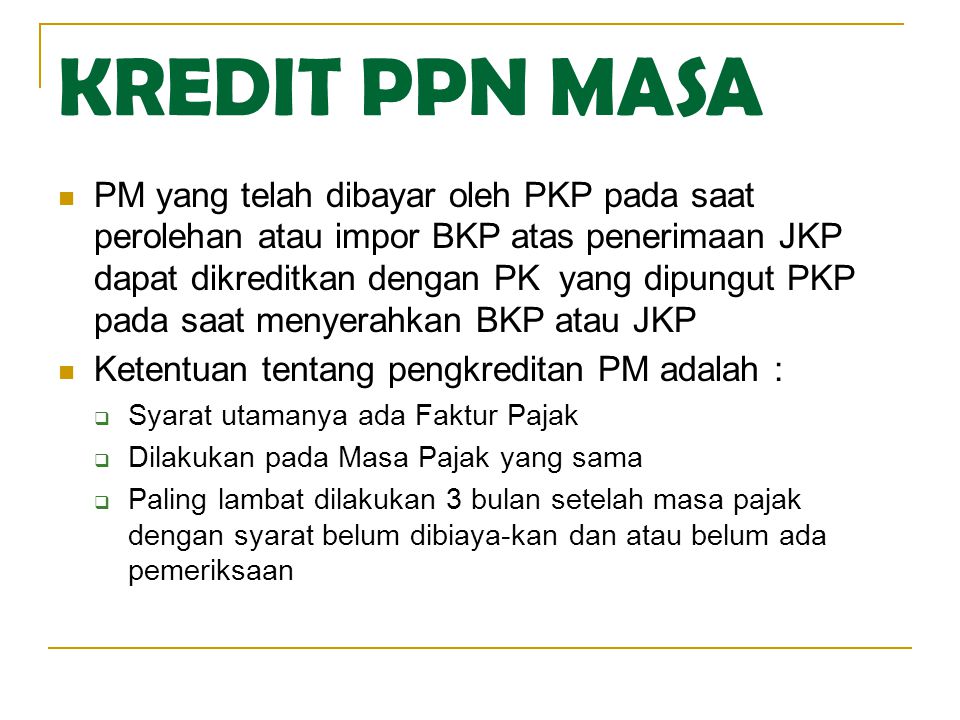This image is a horizontal rectangular slide with partial borders, featuring a yellow line at the top, bottom, and a bit around the upper left corner. The slide is titled "Credit PPN Masa" in large green letters at the top, which are prominently displayed. The language used is not English and possibly of Indian or Hindu origin. Below the title, there are two primary bullet points written in black text, each marked with yellow bullet symbols. The second primary bullet point is further elaborated with three smaller bullet points in a smaller black font. These sub-bullet points are marked by green-outlined squares with white centers. The slide seems to be explaining or detailing the content related to the title "Credit PPN Masa."